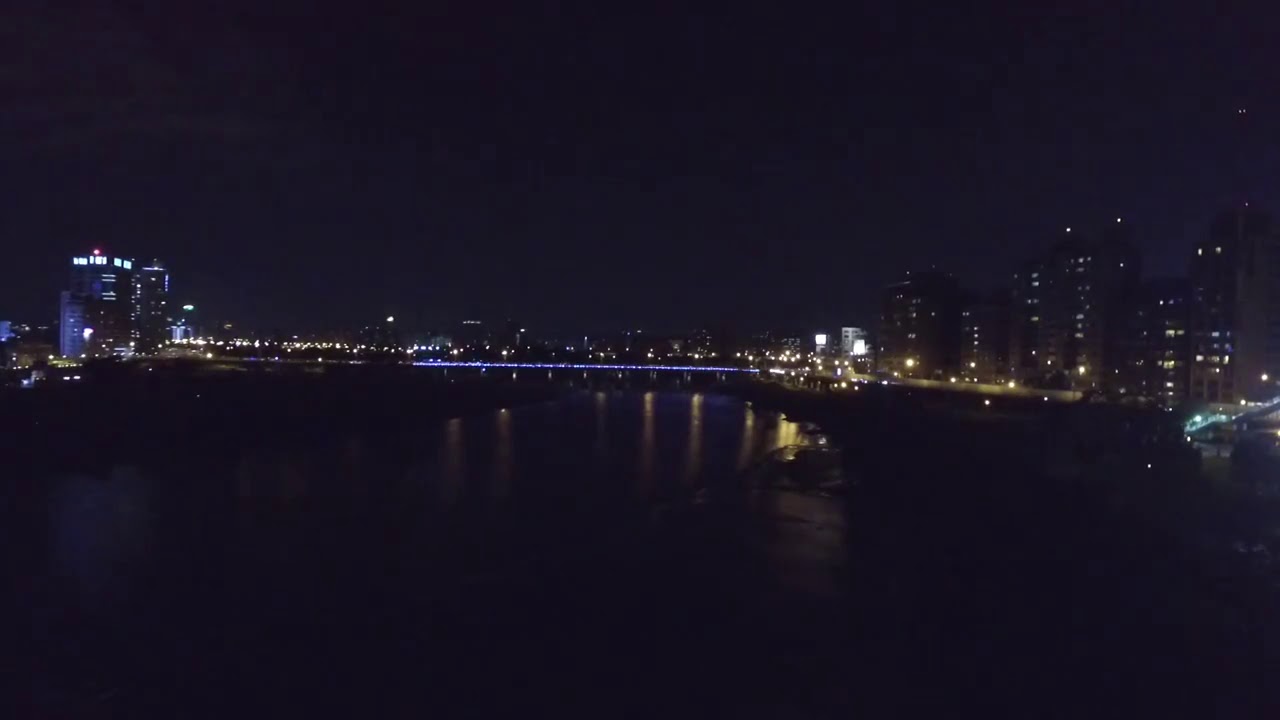The photograph captures a cityscape at night, viewed from above, possibly taken by a drone. The image is anchored by a broad river running horizontally across the middle, bisected by a bridge adorned with a streak of light blue illumination. On either side of the river, tall buildings, ranging from 10 to 15 stories, rise up with their windows aglow, casting reflections onto the dark water below. The left side of the image presents a concentration of these lit structures, which are mirrored by similarly illuminated commercial buildings on the right. Above, the sky is an inky abyss, devoid of stars or the moon, hinting at a cloudy night. Tiny points of light in the top right corner suggest distant airplane or satellite lights. The overall composition, characterized by its realism and representational style, evokes a serene yet dynamic urban nocturne, where artificial lights punctuate the pervasive darkness.